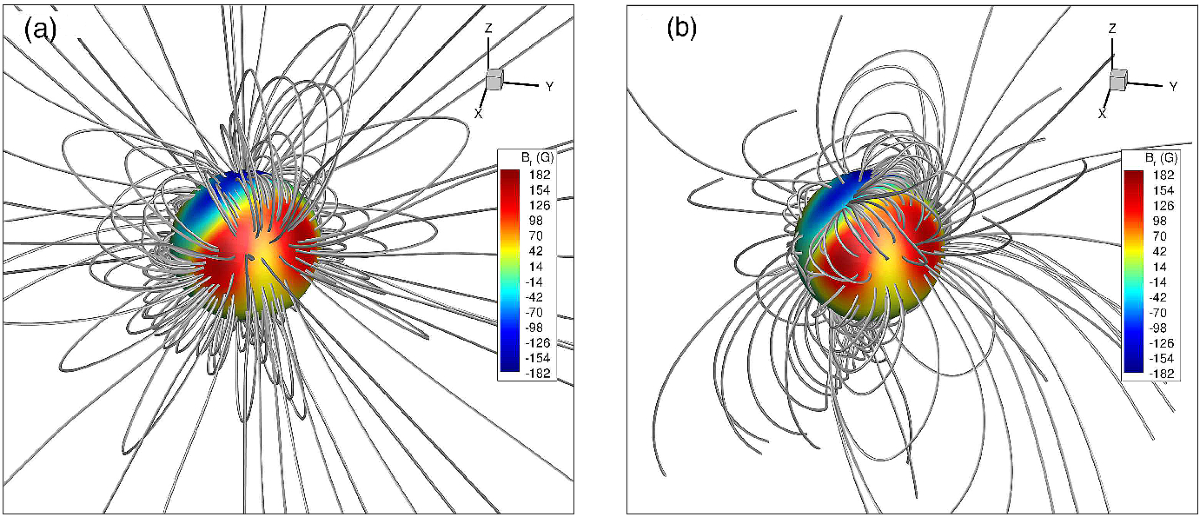The image depicts two adjacent scientific diagrams labeled A and B, each contained within a thin black-bordered square on a white background. Both diagrams feature a central spherical shape that exhibits a swirl of colors, including red, yellow, blue, teal, and green, reminiscent of a partial rainbow (ROYGBIV without violet). The spheres are surrounded by an array of gray lines extending outward in various directions.

Diagram A, on the left, has more numerous and intricately curved lines looping back towards the colorful ball, resembling a tangled knot. This diagram includes a red-to-blue color scale indicating positive and negative values from top to bottom. Diagram B, on the right, displays fewer lines, particularly on its bottom and right sides, while the lines around the top are short and abruptly end. Both diagrams incorporate 3D axis references, with A's lines appearing more organized compared to the relatively chaotic distribution in B.